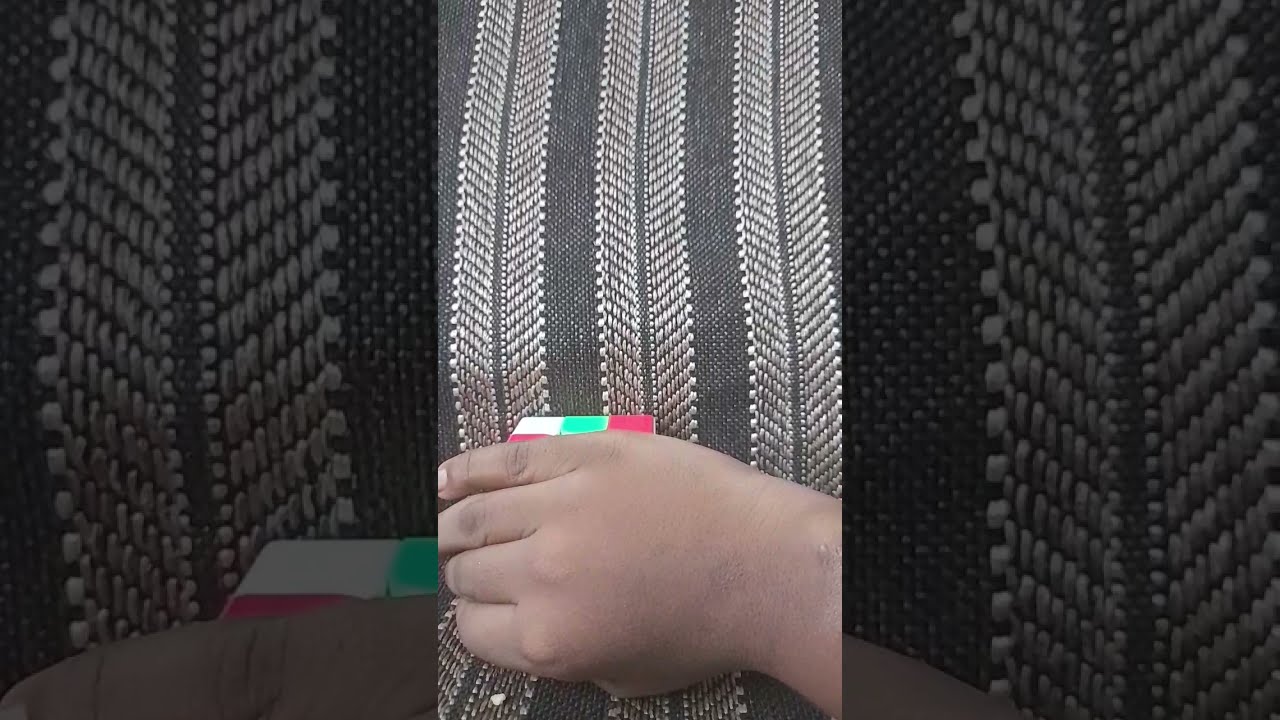A detailed image showcases a brown-skinned hand emerging from the right side, the fingers extending toward the left. The hand, its wrinkles faintly darkened with hints of black, clutches a cube that prominently displays three small squares: one white on the left and one green and red on the right. The cube, which bears a resemblance to a Rubik's Cube, is nestled on a textured surface resembling a woven poncho, adorned with patterns of grey and dark grey lines interspersed with lighter grey, tiny diagonal line patterns. The material is divided into sections, creating a visual impression of an artistic, stylized photo likely manipulated or edited. The unique composition and the positioning of the hand over the cube evoke a sense of depth and layered texture, possibly depicting an individual of African American or Hispanic descent interacting with the object in a staged yet visually compelling manner.